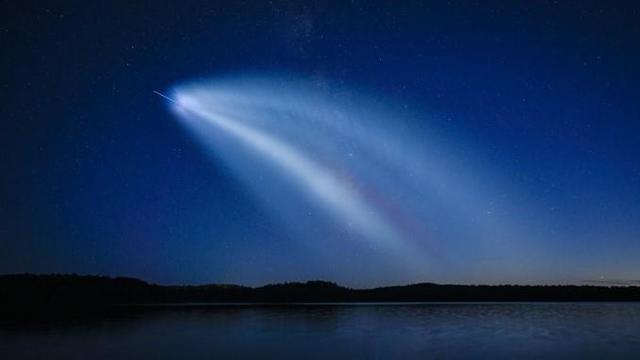The photograph, taken at night, captures a serene lakeside scene. The calm, dark waters of the lake, occupying the lowest portion of the image, reflect the faint starlight from above. A silhouetted, black tree line frames the horizon, with no discernible details due to the lack of light. The expansive sky, which consumes about 75% of the photo, is a deep bluish-black and dotted with distant stars. Dominating the sky is a striking phenomenon: a bright burst of white light emanating from what appears to be a small rocket ship on the left-hand side. The rocket, slender and long, is in mid-launch, trailing a vivid, curving stream of white exhaust. This trail extends from the ground up towards the upper left portion of the image, almost resembling a falling star. The detailed exhaust trail, possibly even containing a faint purple hue, adds a dynamic element to the tranquil scene below. The overall image might have a vignette effect, subtly drawing focus to the celestial activity in the center.